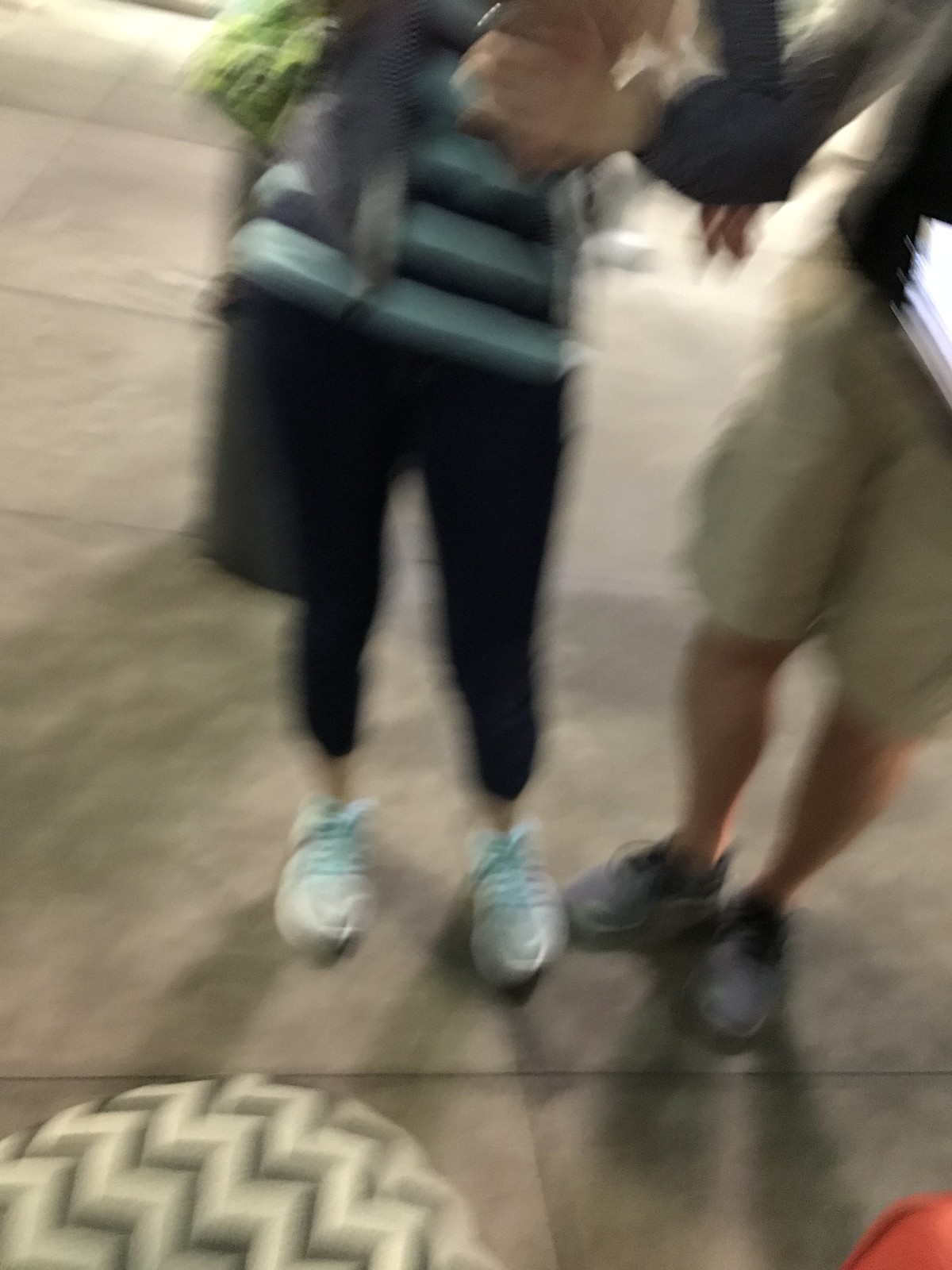This is an extremely blurry photograph capturing the bottom halves of two people standing on a broad gray sidewalk, visible from about mid-chest down. The person on the left is dressed in a horizontally striped blue and black shirt, black leggings, and white tennis shoes with teal laces, also carrying a green bag over their left shoulder. Meanwhile, the person on the right, a man, is wearing a dark-colored long-sleeve shirt, khaki cargo shorts, and gray tennis shoes, displaying notably thick calves. In the foreground, a partially visible round object with a white and gray zigzag pattern can be seen in the lower left corner, while a small red rounded shape is discernible in the bottom right corner, adding further ambiguity to the image.